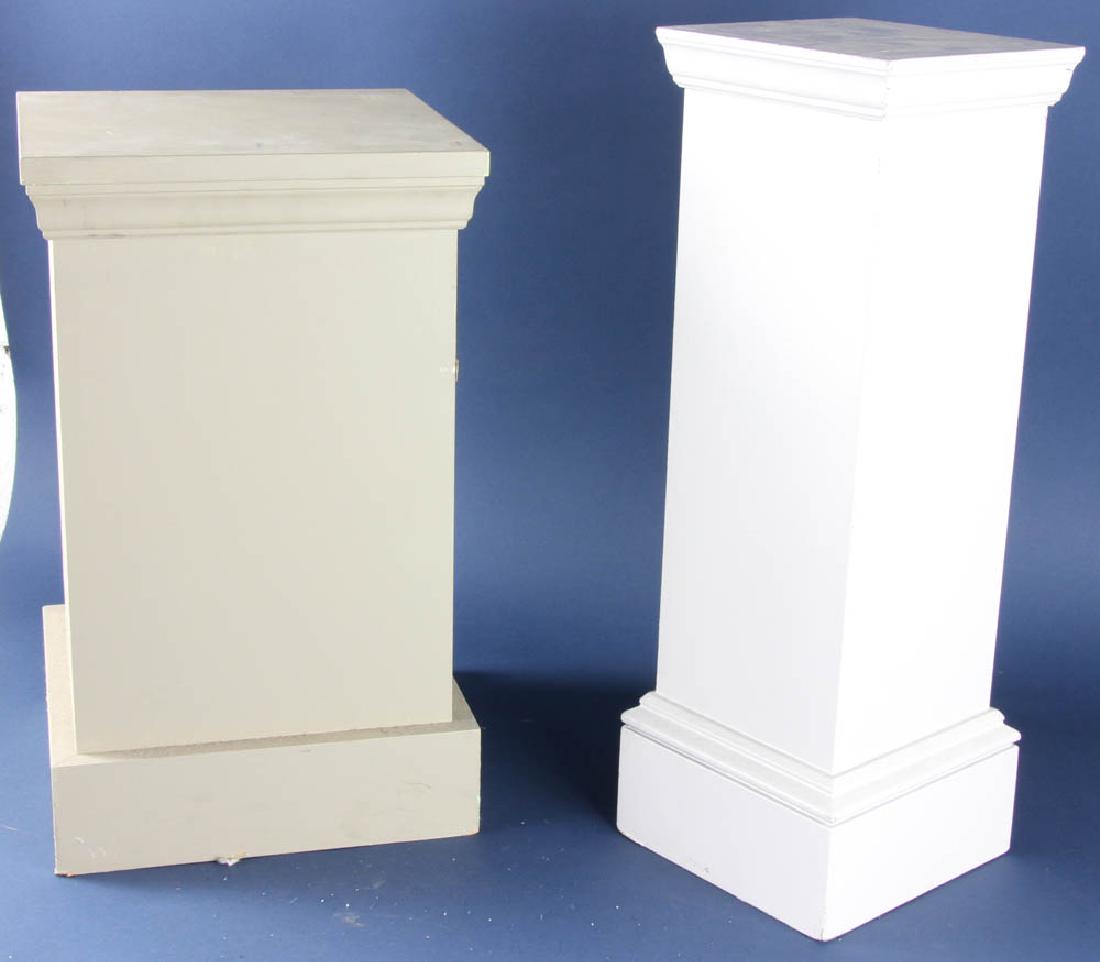The image depicts two upright rectangular pedestals with a Greek-inspired design, standing on a blue floor against a blue background, likely taken inside a studio. The pedestal on the left is off-white, shorter, and wider, featuring an ornate trim around the top and a wider, simpler trim at the bottom. The pedestal on the right is taller, skinnier, and a solid white color, with trim around the top and bottom that flares out slightly. Both pedestals appear clean and sharp-angled, designed for displaying objects such as small sculptures or vases, rather than for any practical, functional use. The overall scene has a minimalistic yet elegant feel, suitable for showcasing art or decorative pieces.